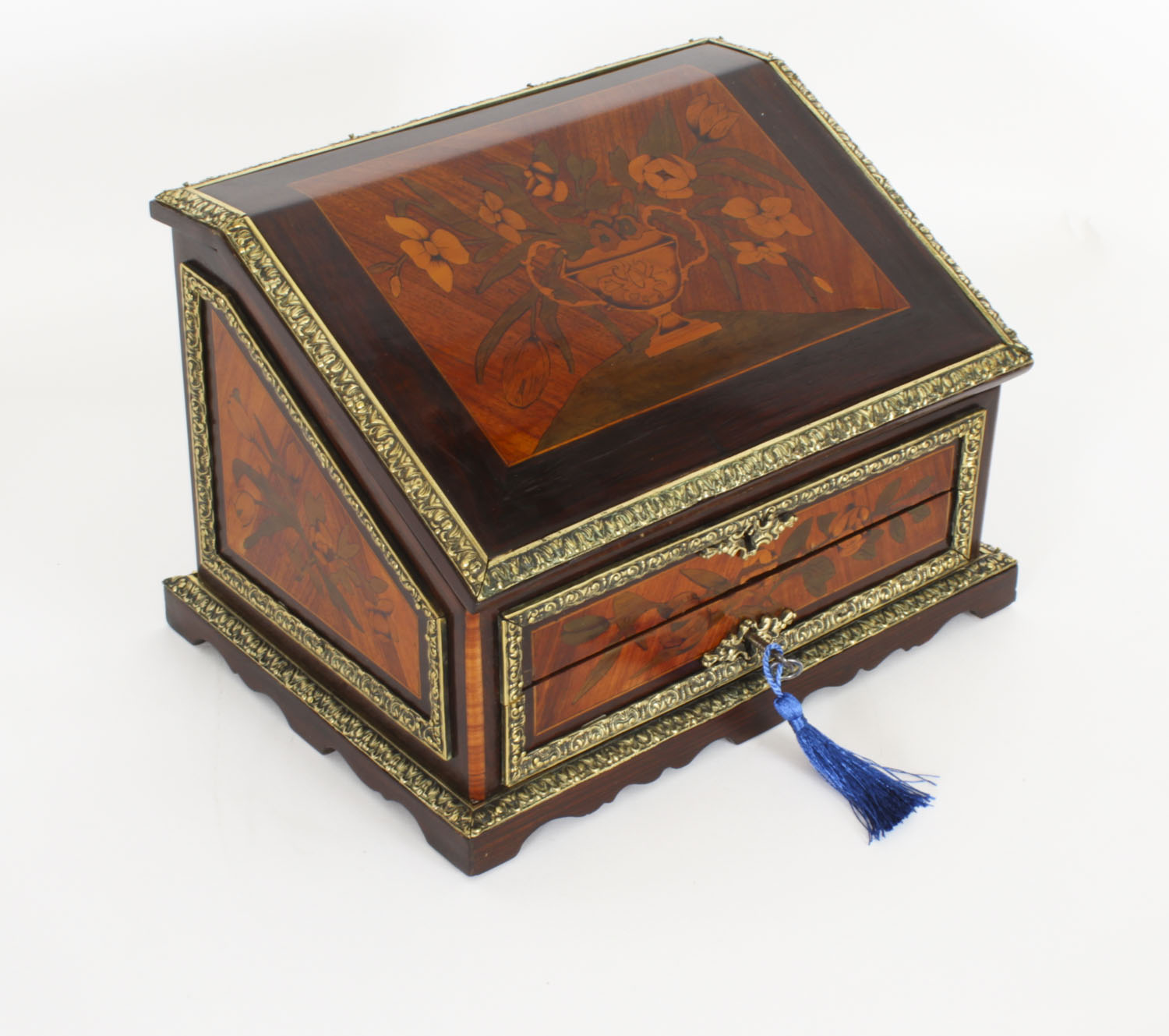This image depicts an ornate, antique-style jewelry box set against a white background. The box is crafted from dark wood with intricate inlays of lighter wood creating a decorative design. The most striking feature on the top is an inlaid image of a vase with large green leaves and small white flowers. This vase design is crafted with remarkable detail, using various shades of wood to create a realistic portrayal of a flower arrangement. The box has a gold trim that outlines its edges, adding to its opulent appearance. The front of the box features keyholes, one of which has a key inserted, adorned with a blue lanyard or tassel. The jewelry box also includes a lift-up lid and two drawers, emphasizing its functionality. This elegant piece appears to be angled slightly away from the camera, offering a glimpse of its intricate details and structure.